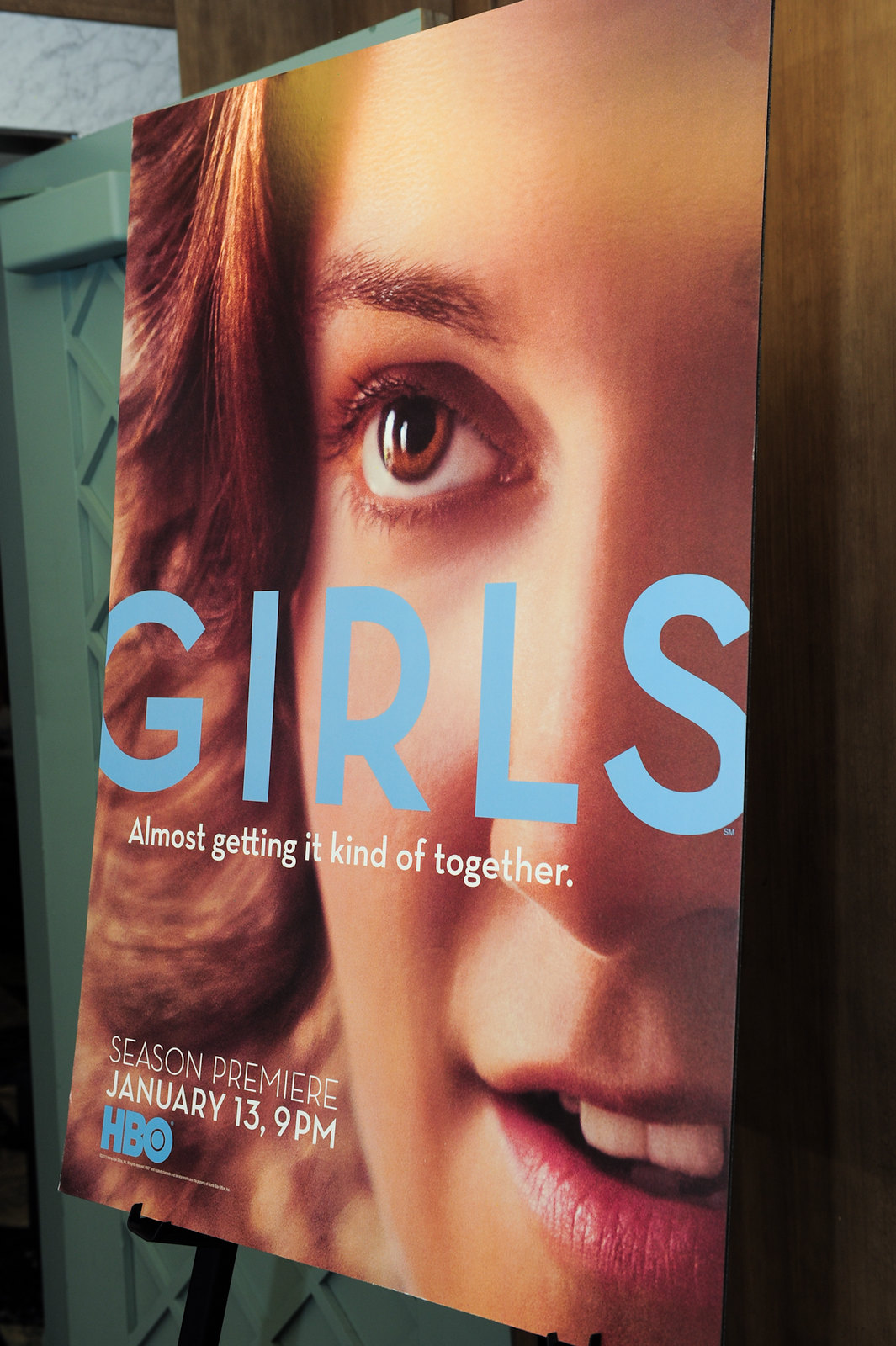This is a full-color photograph of a promotional poster for the HBO show "Girls" set against a backboard or an easel. Dominating the poster is a close-up image of a young white woman's face, likely in her 20s, with hazel eyes and brown curly hair cascading down the front. The word "GIRLS" is boldly printed in large, bright blue capital letters across the midsection of her face, partially covering her cheeks and nose. Below this, in smaller white text, is the tagline: “Almost getting it kind of together.” In the lower left-hand section of the poster, details of the show's premiere are provided: “Season Premiere January 13, 9pm, HBO” in capital letters. The background primarily features the woman’s face, and there is an obstructing dark brown strip, possibly part of the easel or frame, on the right-hand edge of the image. The left side of the frame shows a section of green fencing with lines running through it. This poster appears to be part of a marketing effort for the series "Girls" airing on HBO.